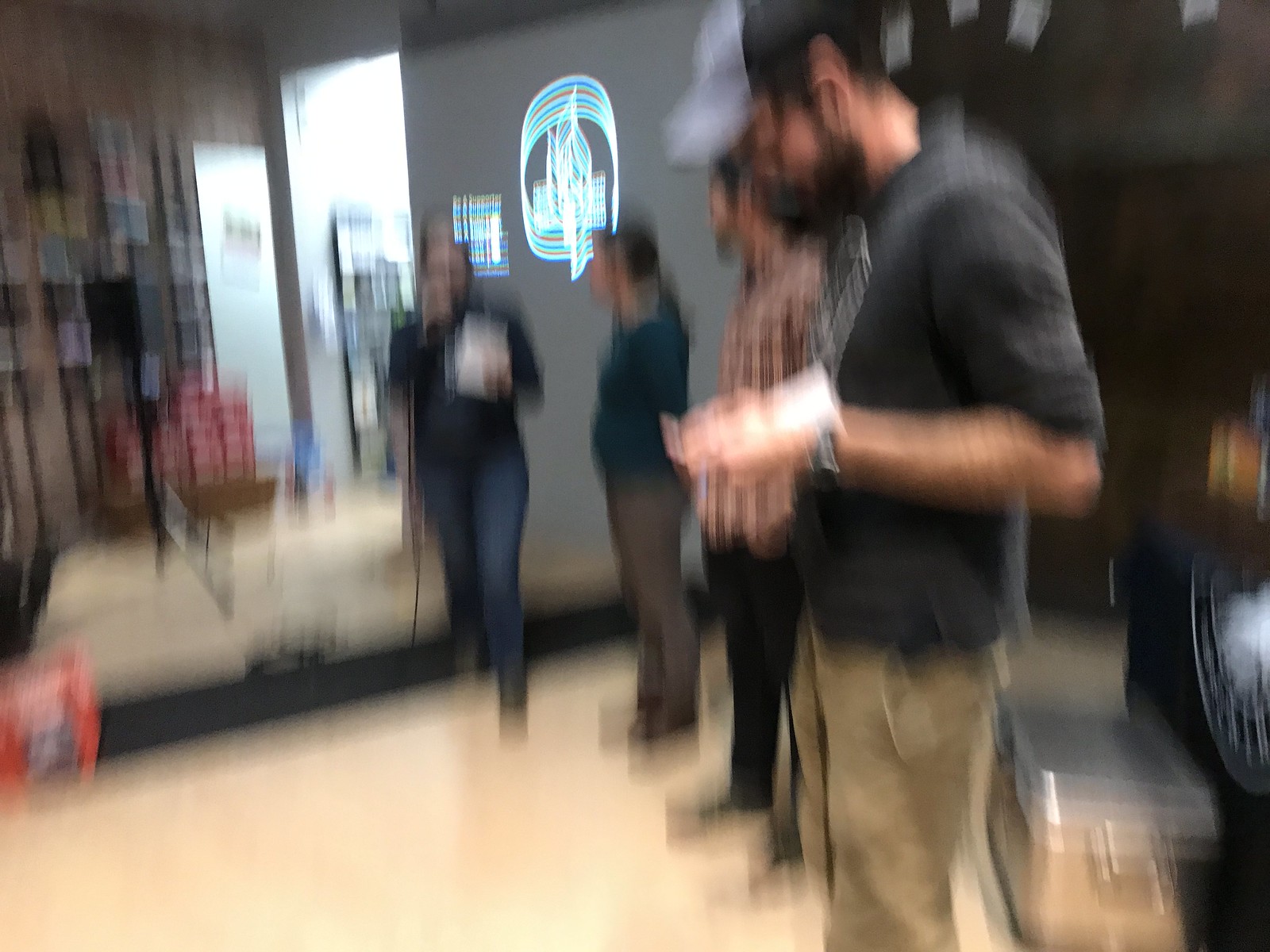In this blurry, out-of-focus photograph, a group of four people stand near a cooler on a reflective, light-colored floor. In the foreground, a man wearing a dark shirt with rolled-up sleeves, khaki pants, a black-and-white baseball cap, glasses, and possibly a beard looks down at an object in his hands, perhaps a piece of paper or a bag of popcorn. To his left stands a bearded man clad in a plaid shirt and dark pants, partially turned towards a woman next to him. The woman, with her hair in a ponytail, is dressed in a green shirt and dark pants and is focused on another woman stepping down from an upper platform. 

This second woman, identifiable by her curvy shape, wears jeans and holds a white item, possibly a bag, in her left hand. She appears to have a cord trailing behind her. A bright blue and white neon sign on a grayish wall can be seen in the background, along with a doorway emitting light, adding depth to the scene. The platform behind them might house racks of pamphlets. The entire setting is hard to classify, adding to the mysterious ambiance of the snapshot.